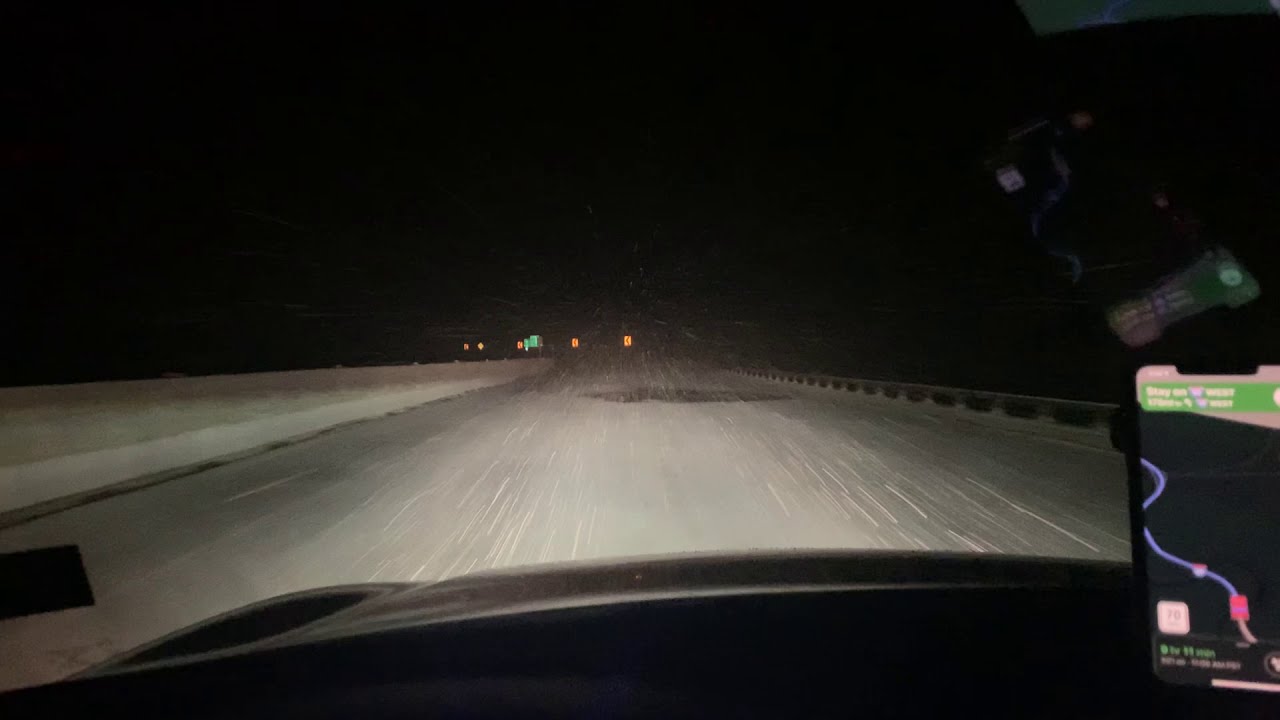The image, captured from the dash cam of a car driving at night, depicts a snowy, deserted road extending into the darkness. At the bottom of the wide rectangular frame, the glossy, curved black hood of the car is visible, emphasizing the vehicle's perspective. In the bottom right corner, a mobile phone mounted on the dashboard displays a GPS map, showing a detailed route with a red car icon traveling along a light blue road. The phone's screen features key navigational cues, including a green rectangle at the top that reads "stay on" with a route icon and the direction "west," alongside a purple squiggly line leading to a pink rectangle marking the destination. Reflecting in the windshield above the phone is a faint image of the same screen, illustrating the interaction of the device with the vehicle's interior.

Ahead, the headlights illuminate the snow-covered highway, revealing dashes of snowflakes cascading towards the car. The road, flanked by a metal railing and a snow-laden embankment on the left, stretches into the pitch-black sky, where distant yellow lights punctuate the horizon. Road signs visible in the distance suggest an upcoming curve, adding to the scene's navigational context. The image, devoid of other vehicles, captures the isolation and stark beauty of a night drive through a snowy landscape.